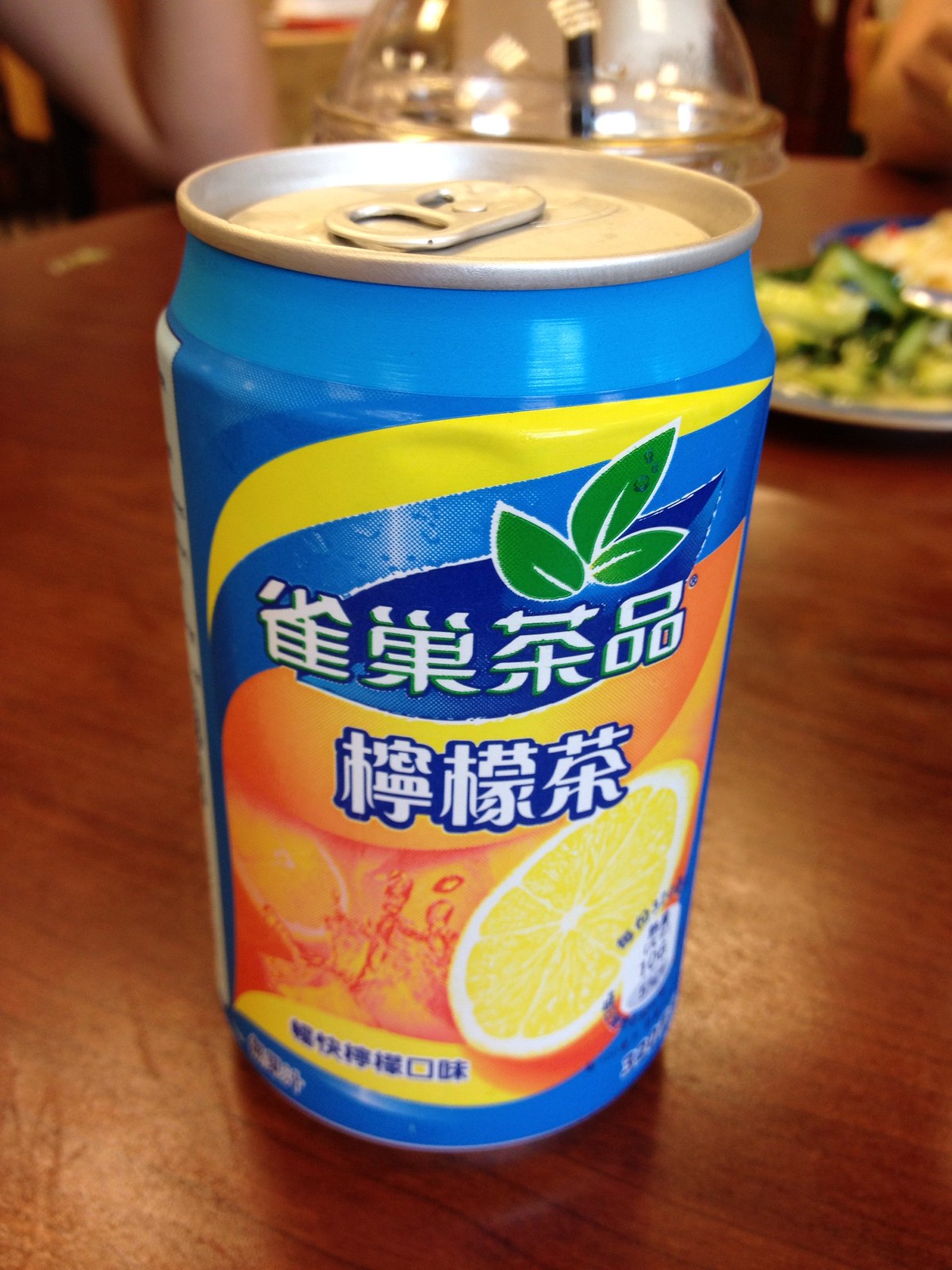This vibrant image showcases a close-up view of an unopened aluminum can adorned with intricate foreign writing, prominently featuring Chinese characters. The can itself is visually captivating with a bright blue base color, accentuated by a striking yellow streak along the top. Just below the streak, three mint green leaves offer a pop of freshness.
 
The main body of the can is predominantly orange, harmonizing with the scattered orange slices artistically displayed on its surface. At the top of the can, a shiny silver snap-type flip-top lid hints at its refreshing contents. The can rests on a smooth, brown wooden table that contrasts beautifully with its vivid colors. 
 
In the background, slightly blurred, there are several items hinting at a laid-back dining setting. Directly behind the can is what appears to be another drink, this one in a cup with a clear plastic lid. To the right of this drink is a plate filled with vibrant green broccoli and a creamy-looking macaroni and cheese dish. On the left side of the image, part of a white arm is visible, adding a subtle human element to the scene.